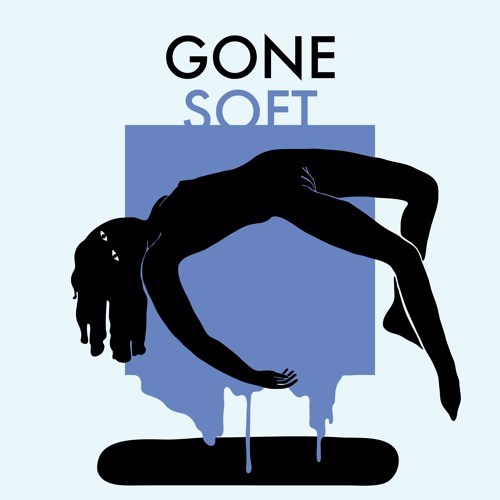The image is a detailed graphical design set against a very light blue background, featuring various elements that come together to form a visually striking composition. Dominating the center of the image is a blue square that appears to be melting towards the bottom, creating the illusion of dripping paint or liquid. This dripping effect merges into a black puddle at the very bottom of the image. Draped over the small blue square is a black silhouette of a woman, depicted with white eyeballs prominently standing out against her all-black form. Her body is arched back, head leaning to the left with her feet extending to the right, giving the impression of her floating or being suspended in mid-air. Above these central elements, the text "Gone Soft" is displayed in two lines; "GONE" in black capital letters and "SOFT" in the same blue as the square. This meticulous design, with its juxtaposition of colors—light blue, black, dark blue, and white—and the melting square, suggests a company logo or something suitable for a business card, evoking a sense of fluidity and surrealism.